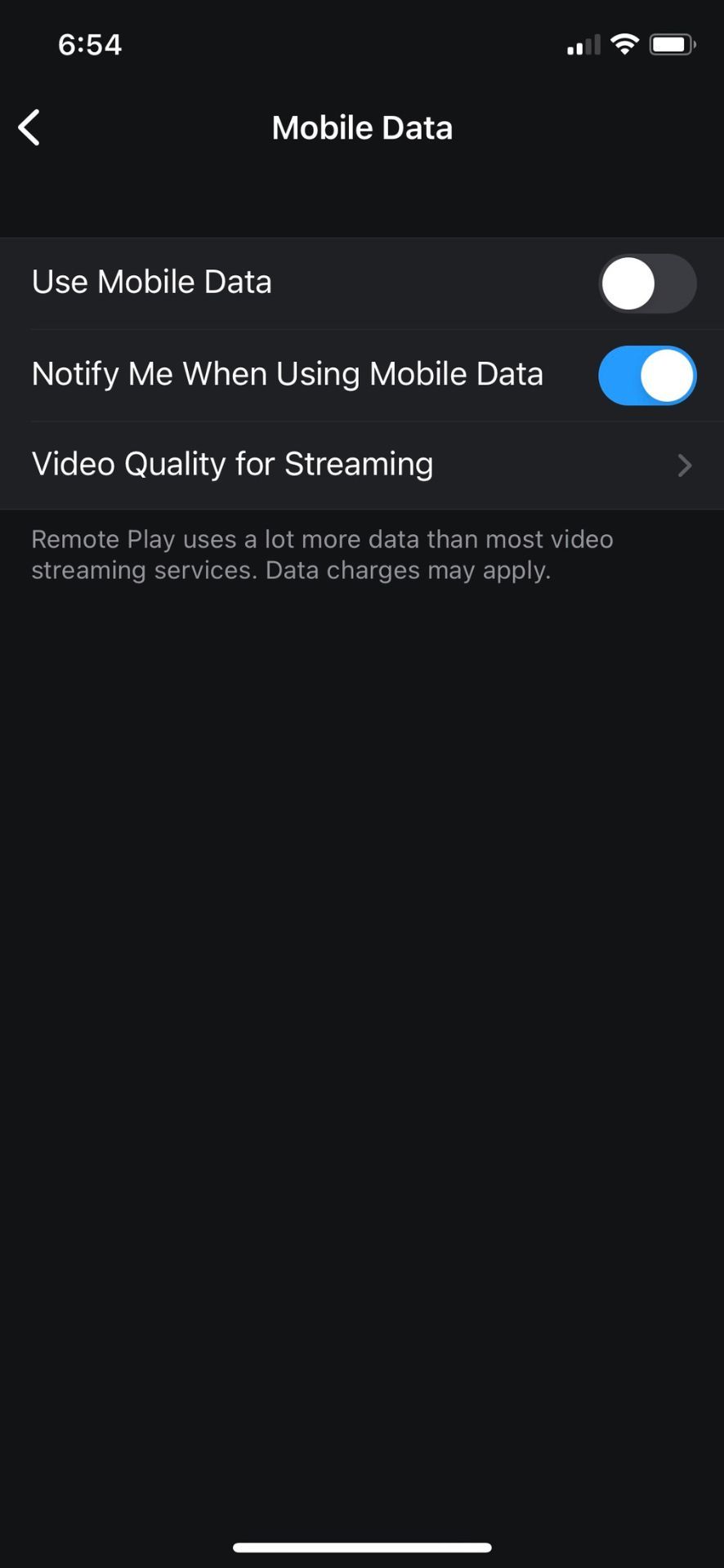A cell phone screenshot features a black background with various interface elements displayed. In the upper left corner, the time is shown in white as "6:54." On the right side, the reception signal, Wi-Fi, and battery icons are visible. 

Centered in gray text, about three lines below the icons, is the label "Mobile Data." To the left of this label is a left-pointing gray arrow, resembling a sideways "V."

Below this section are several dark gray rectangles with white text inside them. The first rectangle on the left reads "Use mobile data," accompanied by a toggle switch on the right. The circle of this toggle switch is white, indicating it is in the 'off' position.

The second rectangle displays "Notify me when using mobile data," with a toggle switch on the right that is turned on. The toggle switch background is aqua, indicating the 'on' position.

Further down, the label "Video quality for streaming" appears, with a right-pointing arrow (resembling a sideways "V") instead of a toggle switch.

At the bottom of this section, in small gray print, there is a warning: "Remote play uses a lot more data than most video streaming services. Data charges may apply."

Centered at the very bottom of the screenshot is a horizontal white line.